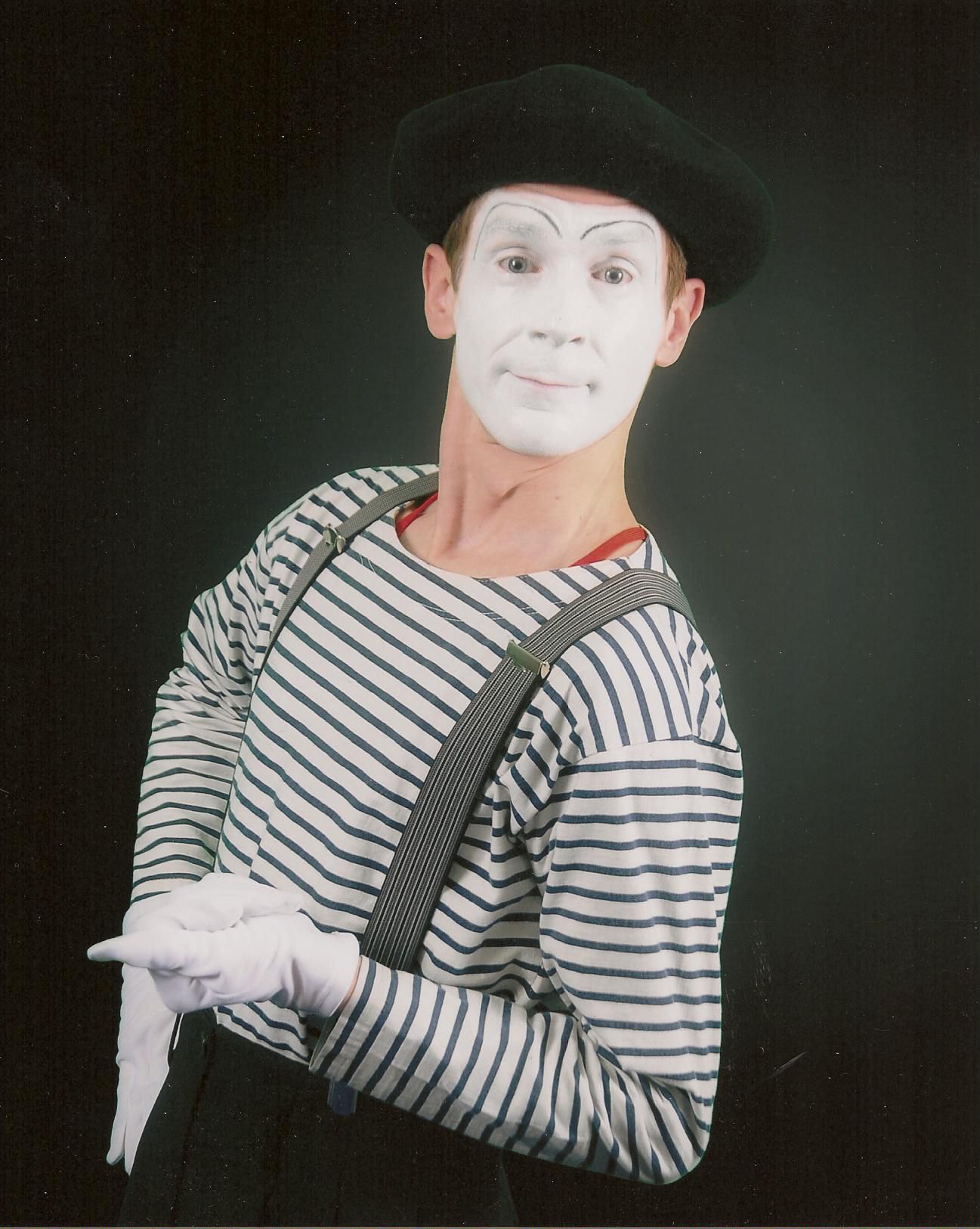The image captures a male mime with white face paint, adorned with thin, high-arching black eyebrows. He is wearing a small black hat over his short brown hair and has gray eyes that directly engage with the camera. His attire consists of a white long-sleeve shirt with narrow, horizontal blue stripes, paired with gray suspenders featuring black and white stripes. He is also dressed in black slacks and white gloves, which accentuate his expressive hand gestures. The mime's body is tilted slightly left in the frame, with his right arm resting on his hip and his left arm bent at a right angle, thumb pointed outward in a dramatic pose. The background is ambiguous, appearing as either a black curtain or wall, adding to the indoor setting's theatrical ambiance. There’s a hint of something red underneath his shirt, yet it's unclear what it is. Overall, the mime appears alert, deeply engaged with the viewer, creating a striking and dynamic impression.